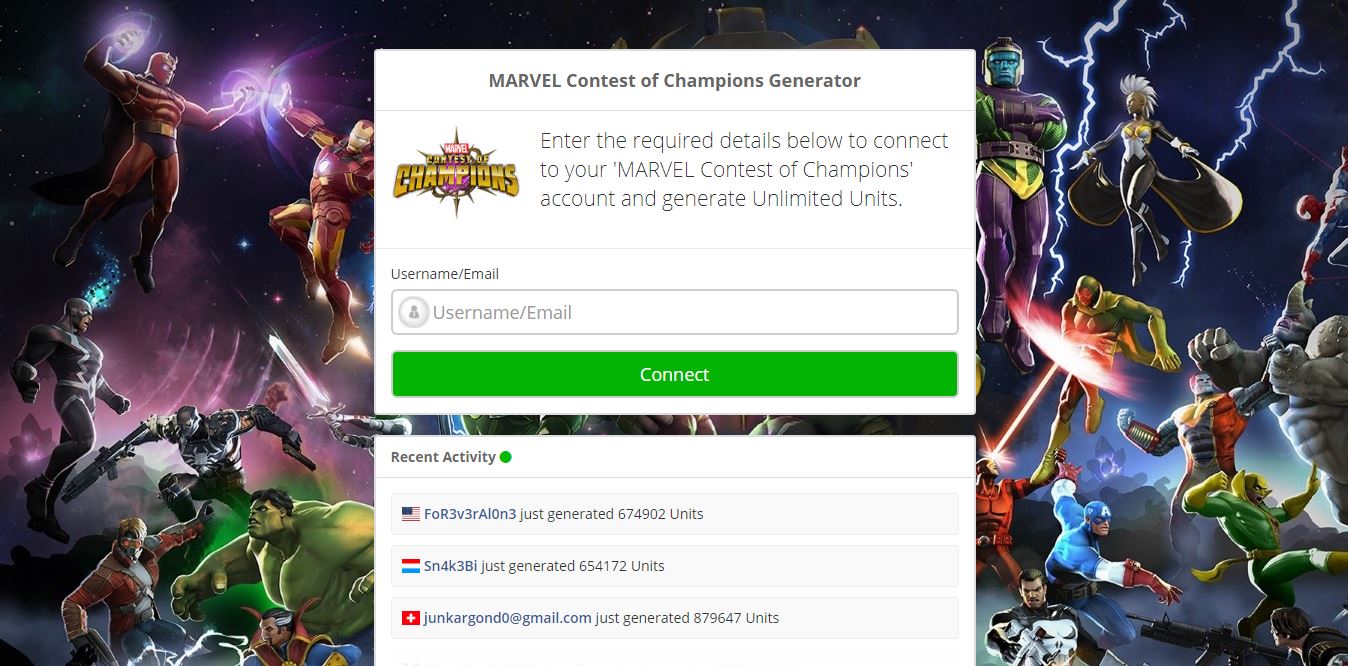In the image, the top section prominently displays the title "Marvel Contest of Champions Generator" in bold, large, and eye-catching text. Below this, a paragraph provides instructions: "Enter the required details below to connect to your Marvel Contest of Champions account and generate unlimited units." It features the Marvel logo, followed by an illustrious, golden "Contest of Champions" title, adding a sense of grandeur to the interface.

Beneath the instructions, there's a user input field labeled "Username/Email," accompanied by a conspicuous green "Connect" button. Directly below this section, the image showcases a "Recent Activity" feed, marked by a green dot symbolizing active status. This feed lists various user-generated actions, including usernames and the impressive number of units they’ve generated. Notable entries include "forever alone," who just generated 674,902 units, "snake bi," and "junk argon...@gmail.com," also generating substantial unit amounts.

The background is a lively illustration featuring an array of Marvel characters engaging in a dynamic battle. Icons like Iron Man, Hulk, the Guardians of the Galaxy, and Captain America are vividly depicted amidst a dramatic, space-themed backdrop, accentuated by striking lightning bolts on the right-hand side, adding to the electrifying atmosphere.